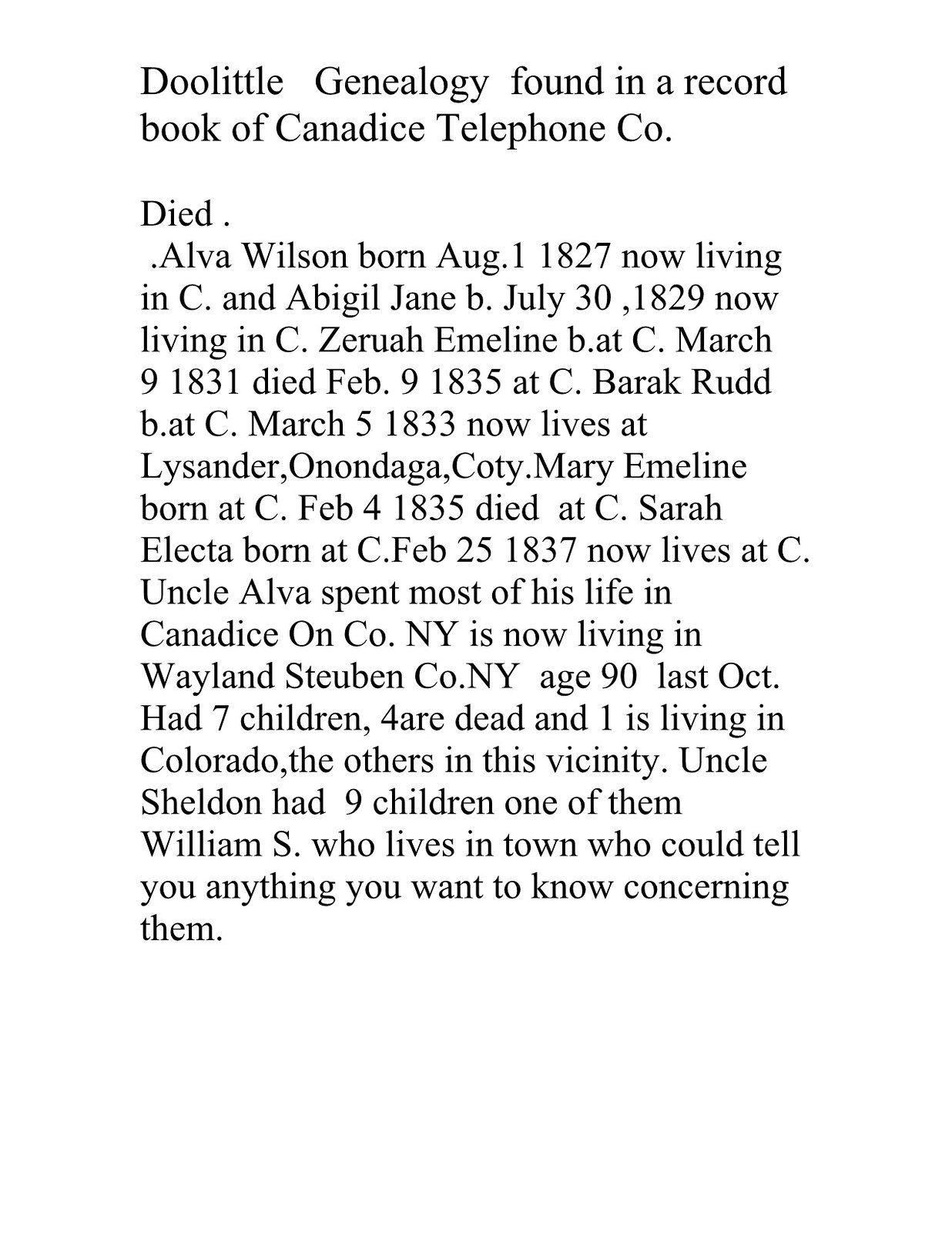The image features a detailed genealogy record against a white background with black text. At the top, it reads "Doolittle genealogy found in a record book of Candace Telephone Company." Below that, the entry details specific individuals: Alva Wilson, born on August 1st, 1827, is mentioned as "now living"; Abigail Jane, born on July 30th, 1829, is also noted as "now living"; Zura Emmeline, born on March 9th, 1831, died on February 9th, 1835; and Barak Rudd is recorded as now living in Lysander, Onondaga County. The image resembles a page from a genealogical search, presenting historical familial data succinctly.